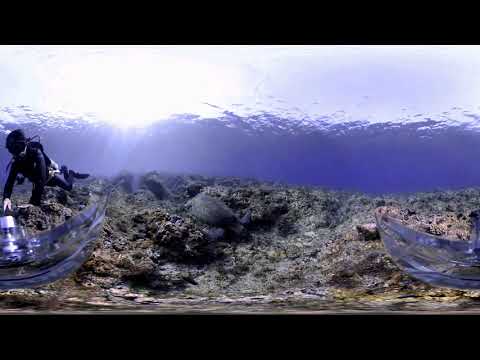This panoramic underwater photograph captures a solitary scuba diver, clad in a black wetsuit, positioned on the left side of the image. He is adorned with a full set of diving gear, including an oxygen tank strapped to his back, goggles, and fins, all extending from his pale hand, which clutches a selfie stick. The ocean floor beneath him appears textured and gray, scattered with lumps and isolated patches of smoother sand, giving it a desolate feel with minimal marine life present. On the right side of the image, there is an instrument resembling a wing structure, which the diver is holding in his right hand. Notably, a shaft of light penetrates the water from the upper left corner, casting a sun flare through the water and creating a play of light that enhances the scene's ethereal quality. Additionally, there are thick black borders at the top and bottom of the image, framing the scene.